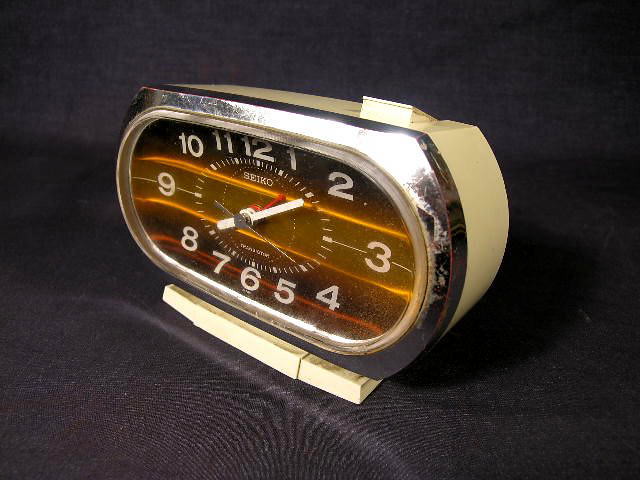This indoor color photograph is a detailed close-up of a vintage alarm clock, likely from the late 1950s to early 1960s. The clock, resting on a black surface with discernible wood grain, is captured in a three-quarter view showing both the front and side. Its oval face, surrounded by a chrome bezel, features a black background with white numbers indicating the time as 12 minutes past 8. The clock hands, including the thin metal second hand pointing to 4, are also white. A red dial, possibly indicating the alarm setting, is present. The clock’s face bears the brand name Seiko (S-E-I-K-O) just below the 12 o'clock position. The cream-colored plastic body, which has aged to a dingy yellowish hue, contrasts with the highly reflective metallic, goldish-yellow bronze surface of the clock face. A prominent button, likely for the alarm, is visible on the top. The overall heavily worn appearance and retro design contribute to its distinct mid-20th century charm.